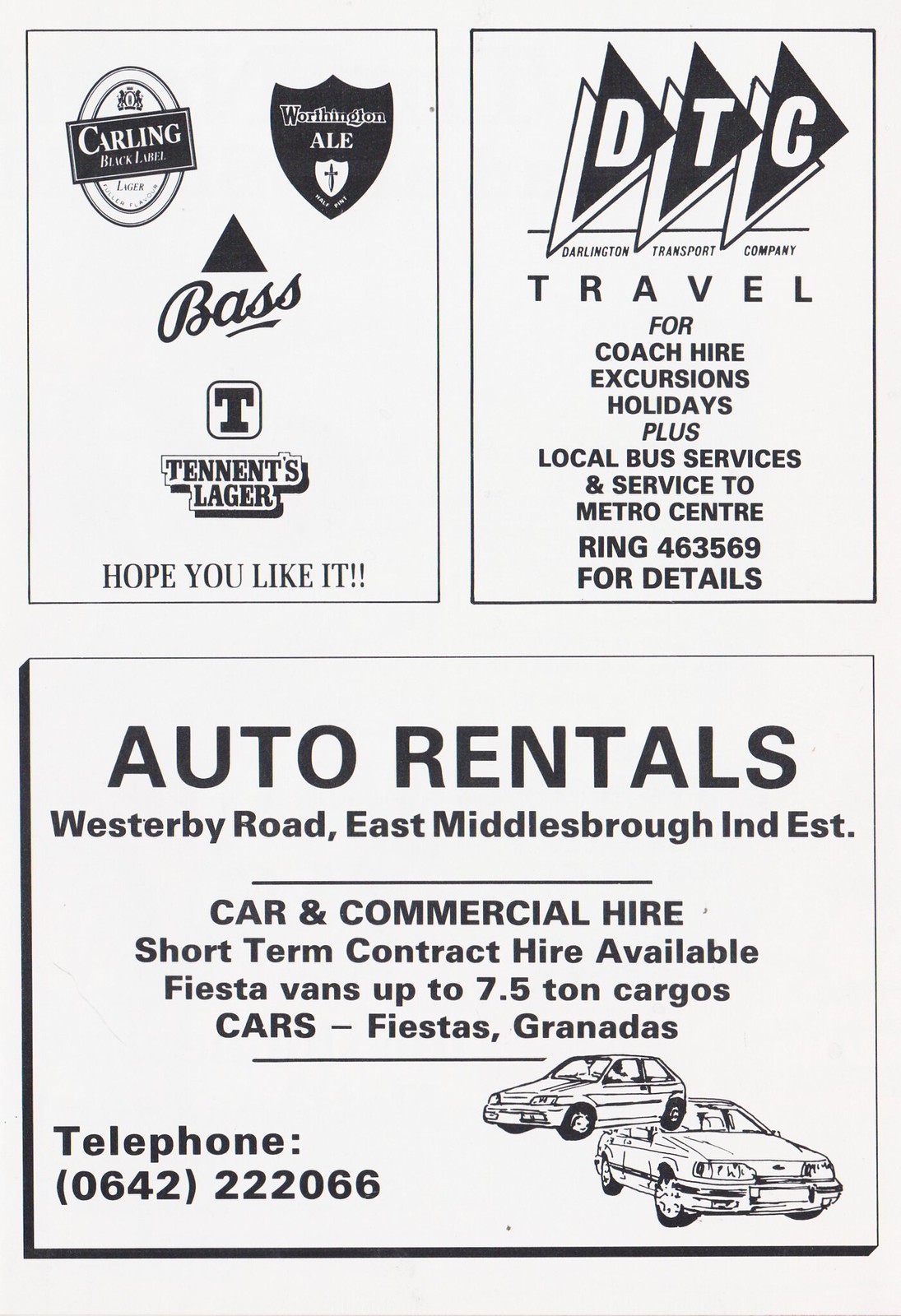In this portrait-oriented image resembling an old newspaper or magazine advertisement page, a pale gray background hosts three outlined sections. The top half features two equal-sized rectangles side by side, while the bottom half consists of one large rectangle.

The top-left rectangle is divided into multiple segments. At the top, there's an oval logo with a black bar inscribed with "Carling Black Label, Lager." Just to the right, a black shield contains the words "Worthington Ale," with a smaller white shield inside that has a sword and the label "half-pint." Below these, the word "Bass" appears in cursive beneath a black triangle. Further down, there is a T symbol within a beveled circle, followed by the text "Tenants Lager." At the bottom of this section, the phrase "Hope You Like It!!" concludes the advertisement.

The top-right rectangle showcases black triangular shapes pointing to the right, above the initials "DTC." Beneath this, the text reads "Darlington Transport Company, Travel for Coach Hire Excursions, Holidays Plus, Local Bus Services, and Service to Metro Center. Ring 463569 for details."

Occupying the lower half of the page, the large rectangle advertises auto rentals. It includes bold text: "Auto Rentals, Westerby Road, East Middlesborough, IND, EST." Below this, it details services: "Car and Commercial Hire, Short Term Contract Hire Available, Fiesta Vans, Up to 7.5 Ton Cargoes, Cars, Fiestas, Granadas." The bottom left corner contains the telephone number "0642-222-066" and to the right, there are illustrations of two cars.